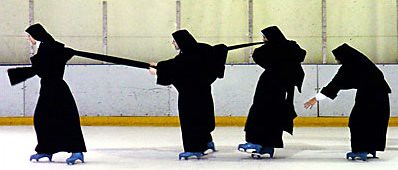This image captures a unique and delightful scene of four nuns ice-skating together on a rink. They are all dressed in their traditional black habits, complete with white collars and veil-like headpieces. The nuns are wearing blue ice skates, which stand out against the pristine white ice. They appear to be gliding in a line, each holding onto the other. The nun at the far right is reaching out, attempting to grab the habit of the nun in front of her, adding an element of playful pursuit. The ice rink features a white barricade with a striking yellow stripe at the bottom, as well as clear glass panels above the barricade, sectioned off as is typical in an ice rink setting. The environment adds to the charm of the scene, with the brightly lit rink devoid of any other skaters, emphasizing the nuns' joyful and serene moment on the ice.